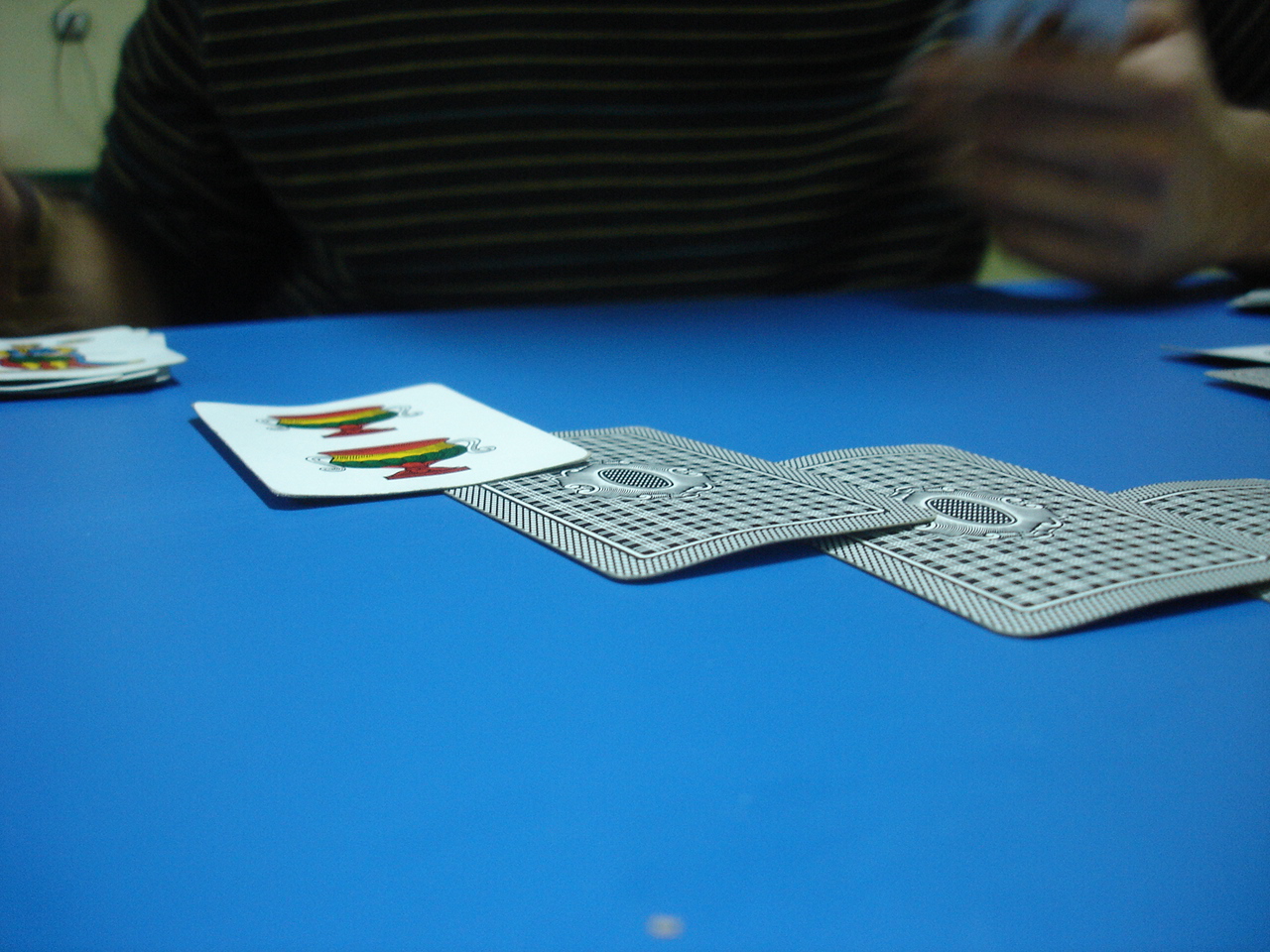A man, visible from his neck to his mid-torso, is engaged in a mysterious card game at a blue table. He wears a dark, short-sleeved shirt adorned with white horizontal stripes. Spread across the table are several cards, the majority of which are face down, featuring a blue-gray plaid checkerboard pattern. Intriguingly, the few cards that are face up are unconventional, with one card depicting an image of two urns rather than a traditional suit. This unique design suggests the possibility of a non-standard card game being played, perhaps something akin to Go Fish. The man has a collection of face-up cards positioned next to him, adding to the enigma of the game. Scattered in the center of the table are approximately seven cards, with only one or two revealing their peculiar face-up details.